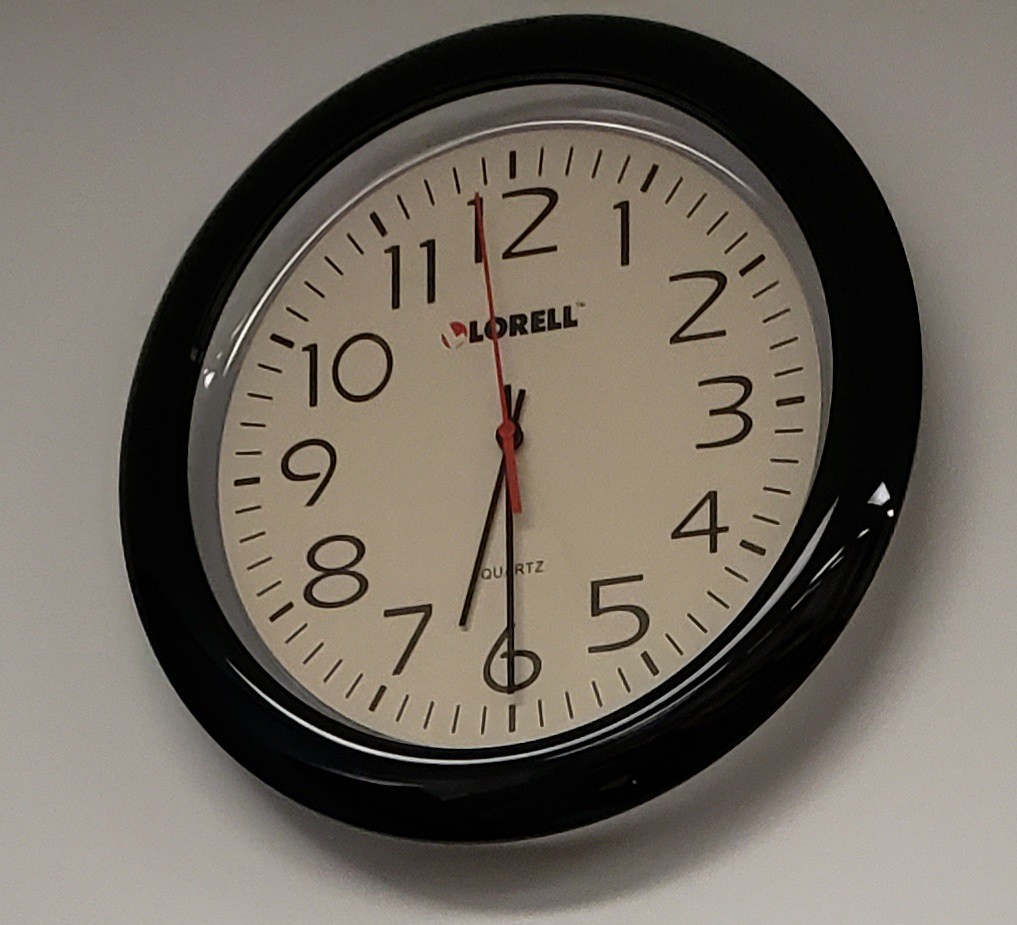The photograph depicts a round analog clock hanging on a pristine white wall. The clock features a shiny black border encircling its face, which is primarily white with bold black numerals. The brand name, "LORELL," is prominently displayed in capital letters right beneath the 12 o'clock position, along with a red circle containing the letter "L". Just above the 6 o'clock position, the word "QUARTZ" is inscribed in smaller lettering. The clock displays the time as 6:30, with a precise red second hand positioned close to the 12. Notably, there is a gray-colored section on the clock face, possibly due to the angle of the photograph, which was taken from a slightly diagonal, lower perspective.